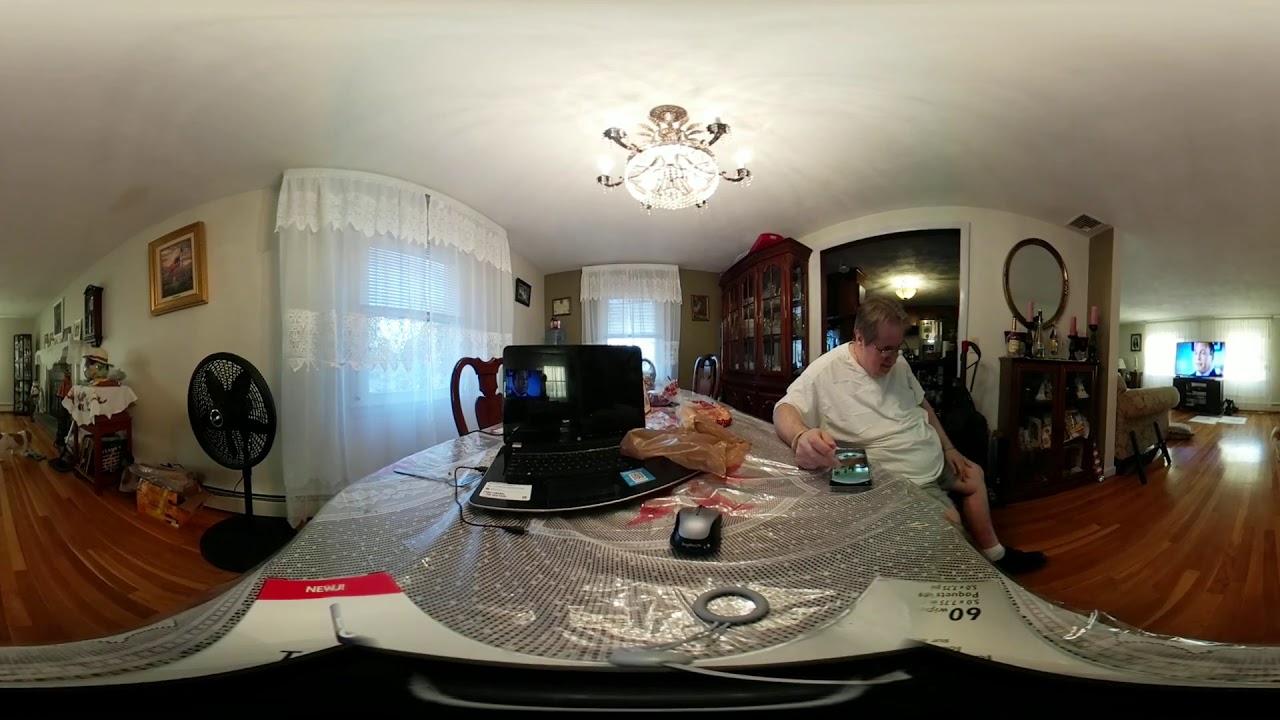In this horizontal rectangular image taken indoors, a detailed kitchen scene is captured. The walls, ceiling, and ceiling light fixture are all white, providing an airy backdrop to the dark brown wooden floor. Dominating the center of the scene is a table draped with a gray and white tablecloth, laden with various items including a black laptop, its mouse, and what appears to be a couple of smartphones. Seated at the table is a person—likely a woman—with short blondish-brown hair and glasses, dressed in a white t-shirt, shorts, socks, and dark shoes. She is looking down, possibly at the floor or the objects in front of her, and holding what might be a coffee cup.

To the left of the table, a black standing fan is positioned near a hallway visible on the far left side of the image. The walls are adorned with various picture frames and mirrors, adding to the room’s decor. Multiple windows draped with sheer white lace curtains allow soft light to fill the space. In the far right background, a television set and part of a likely living room with a touch of a display case and a circular gold mirror on the wall can be seen, adding depth to the image.